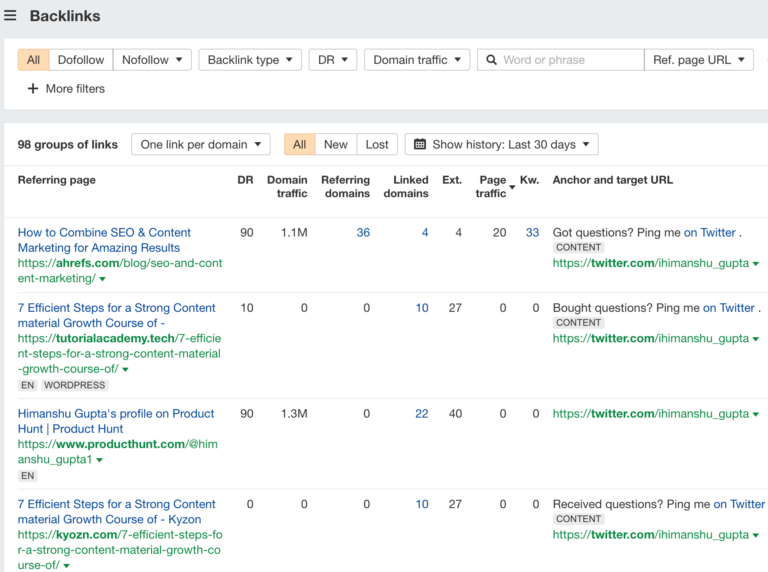Title: Detailed View of a Backlink Analysis Tool Interface

Caption:
The image showcases a sophisticated interface of a backlink analysis tool, designed for SEO professionals. At the very top of the interface is a gray navigation bar with the word "Backlinks" prominently displayed in the upper left-hand corner, accompanied by a three-bar menu icon for additional options.

Below this bar, there is a comprehensive filter menu with several drop-down selections, facilitating refined data analysis. The menu options from left to right include: 
- "All" 
- "Do Follow" with a drop-down menu
- "No Follow" with a drop-down menu
- "Backlink Type" with a drop-down menu
- "DR" (Domain Rating) with a drop-down menu
- "Domain Traffic" with a drop-down menu
- An empty search bar 
- "Referral Page URL" with a drop-down menu.

An additional option is indicated by a plus sign and the words "More Filters," suggesting that more filtering options are available if needed.

Beneath this filter menu is another gray line, followed by a text section indicating "98 Groups of Links" with a drop-down menu defaulting to "one link per domain." Users can further select between "All," "New," or "Lost" links and utilize the "Show History" option, which is currently set to display data from the "last 30 days."

The main content area below this section lists individual backlinks, each entry providing extensive data. Columns include:
- The title of the link
- The actual URL
- Referring Page DR (Domain Rating)
- Domain Traffic
- Referring Domains
- Linked Domains
- Extension
- Page Traffic
- KW (Keywords)
- Anchor text
- Target URL

This layout offers a comprehensive, user-friendly view for in-depth backlink analysis, enabling users to meticulously track and manage their SEO efforts.